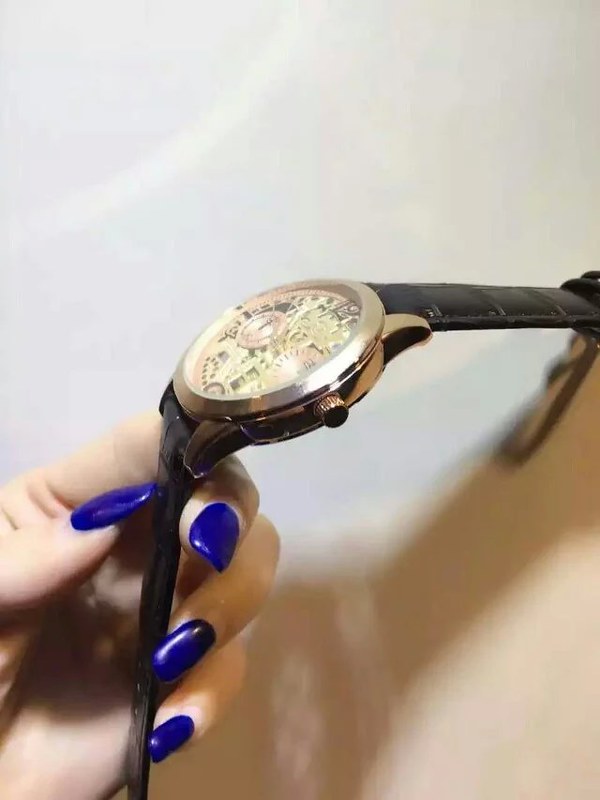A close-up image features a woman's hand delicately holding an elegant watch, prominently showcasing her long, meticulously manicured blue nails. The watch, which she grips in one hand, boasts a striking leopard-patterned leather band that adds a touch of wild sophistication. Its face, rimmed in gleaming gold, reveals intricate mechanics, offering a glimpse into the artistry of its inner workings. An adjustment knob on the side of the watch contributes to its functionality and design appeal.

Shadow and reflection play a subtle role in the visual story, indicating that the woman’s hand, appearing with a hint of flesh color underneath, casts a soft shadow onto the surface below, though the exact nature of the surface remains ambiguous. The backdrop of the image is a simple, beige-colored wall, allowing the luxurious details of the watch and the woman's elegant hand to remain the focal point of this meticulously composed scene.